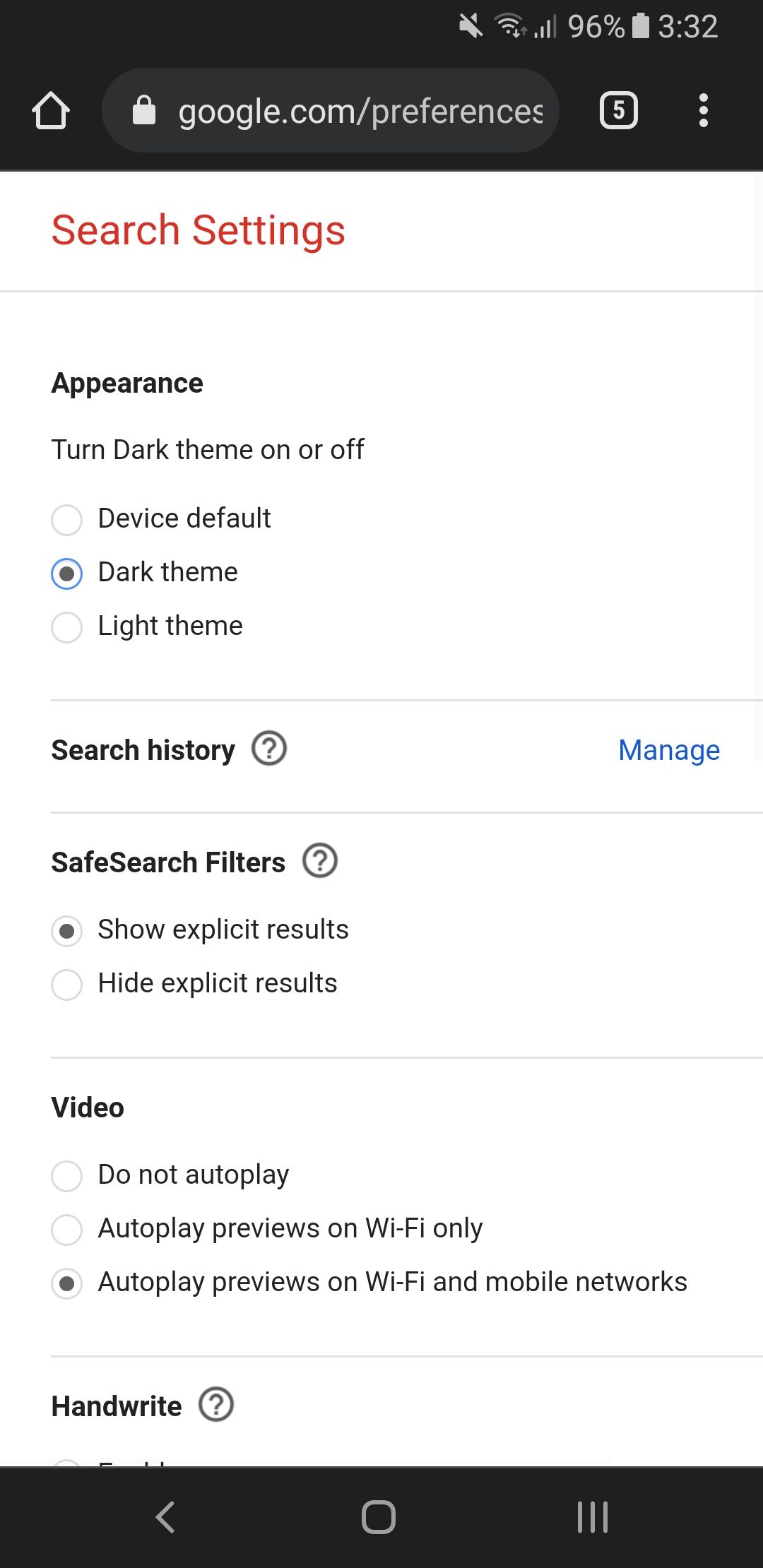The image shows a mobile device screen with a black status bar at the top displaying a 96% battery charge and the time, 3:32. Below the status bar, there is a webpage open with a home button and a search URL box, secured with a lock icon, indicating "google.com/preferences".

The main content area of the page starts with a headline in red text reading "Search settings", followed by a light gray horizontal line underneath it. The first setting, labeled "Appearance," has options for adjusting the theme: "Device default," "Dark theme," and "Light theme," each with a selectable circle to the left. The "Dark theme" option is currently selected.

Below the Appearance section is "Search history," accompanied by a circle with a question mark icon and a clickable blue hyperlink labeled "Manage." Further down is the "SafeSearch filters" section, which also has a question mark icon. This section provides options to "Show explicit results" and "Hide explicit results," each with a corresponding circle to the left. The "Show explicit results" option is selected.

At the bottom, there is a "Video" section detailing autoplay settings with two options: "Do not autoplay" and "Autoplay preview on Wi-Fi only."